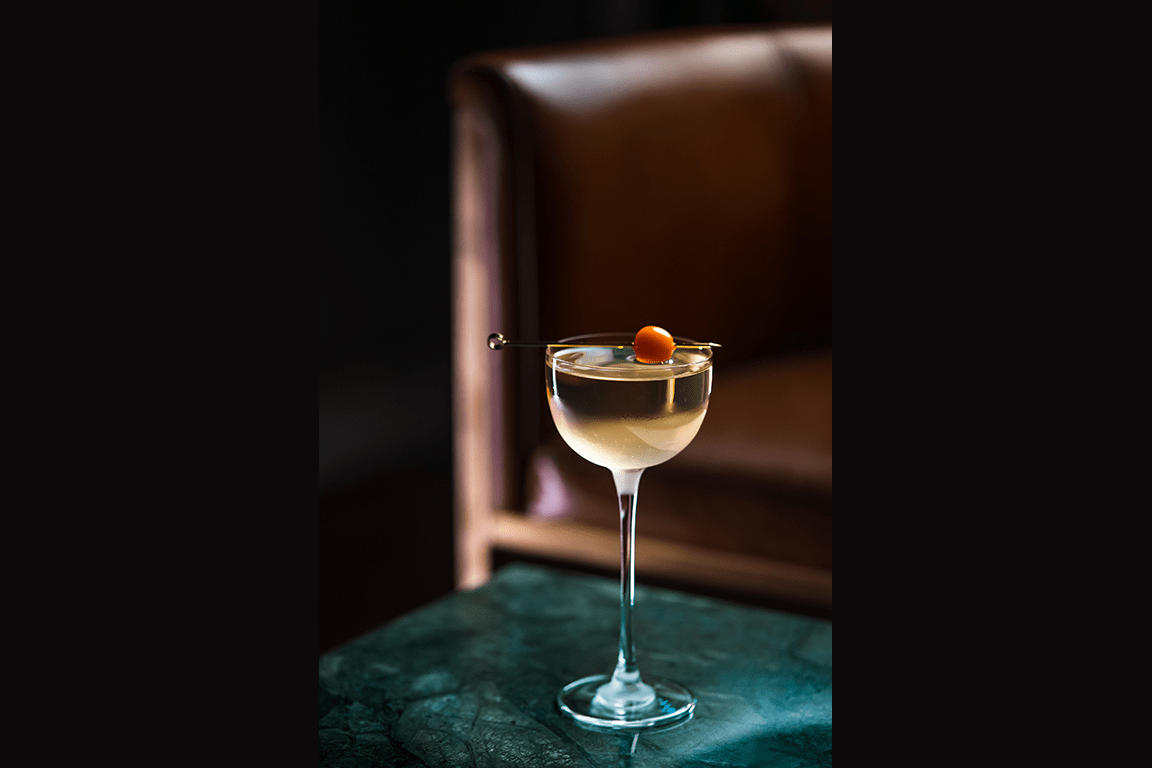This detailed color photo captures a close-up of a martini glass centered on a green marble countertop. The glass, which features a long stem and a wide bowl, holds a clear amber liquid reminiscent of white wine. Laying across the top of the drink is a metal skewer, impaling a red garnish that appears to be a cherry. The scene is illuminated from behind, highlighting the glass and drink while the background remains blurred. The photo is framed by heavily shadowed sides, with dark, indistinguishable elements hinting at a cabinet or chair in the dimly lit room.